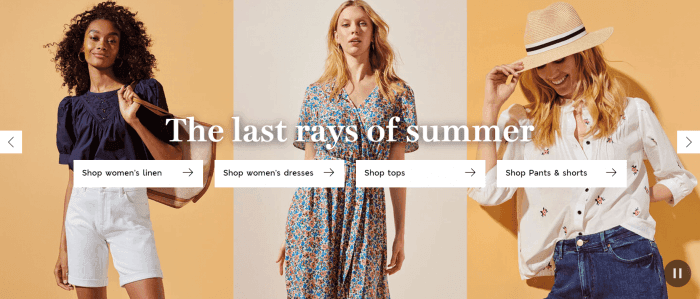The image appears to be an advertisement from a website, featuring three women against different colored backgrounds. 

On the left, an African-American woman with shoulder-length frizzy hair stands against a light orange backdrop. She is dressed in a blue top and white shorts, and she carries a stylish brown and white handbag over her left arm and shoulder.

In the center, against a white background, a blonde woman gazes directly into the camera. She is wearing a blouse adorned with a blue and orange floral pattern.

On the right, another blonde woman, wearing a cap and looking downward, completes the trio. She sports a white button-up shirt decorated with red and blue flowers, paired with blue jeans.

To the left of the woman on the left, an arrow in a little white box points to the left. Similarly, to the right of the woman on the right, an arrow in a little white box points to the right.

The text "Last rays of summer" is displayed prominently across the middle of the image in white letters.

Underneath, near the waistline of the woman on the left, the following shopping options are listed:
- Shop with Lemon
- Shop with Dresses
- Shop Tops
- Shop Pants and Shorts

In the bottom right corner of the image, there is a pause button.